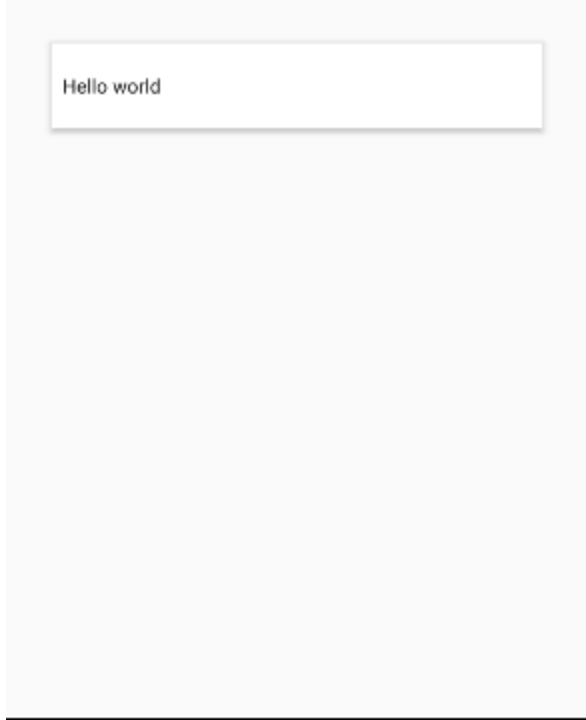This image is a screenshot from an unidentified web page. The screenshot lacks a header or a navigation bar, making it impossible to ascertain the website's address. The footer is also absent, offering no additional clues about the website. The background of the page is an extremely light gray, almost white, providing a subtle contrast. At the top, there is the faint outline of a white rectangle. Within this rectangle, on the left side, the phrase "Hello World" is written in gray font. At the bottom of the image, a dark gray line stretches horizontally across the page, from left to right. Due to these limited elements and the absence of any distinctive features, it is challenging to determine the specific nature or type of the website. However, the phrase "Hello World" is commonly associated with WordPress, as it typically appears as a default post when setting up a new WordPress site.